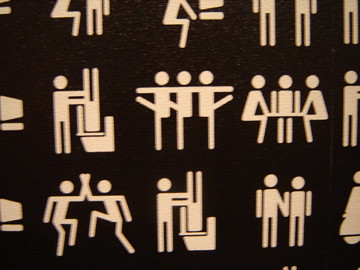The image features computer-drawn, simplified yellow male figures with circle heads on a stark black background, resembling the kind of figures used on bathroom doors to denote gender. The scene is composed in rows, with the top row partially cut off but mirroring the varied poses below. 

From left to right in the detailed bottom row, the first depiction shows a man holding another man upside down, dunking his head into a toilet bowl. Following this, three male figures stand in a line, arms draped over each other's shoulders, executing high kicks akin to the Rockettes. This is succeeded by three figures seated around a table, engaging in a discussion or activity. The next pose features two figures facing each other, engaging in a celebratory high-five. Another image repeats the depiction of one man dunking another’s head into a toilet bowl. Finally, two figures are shown side by side, with one figure resting a hand on the other's shoulder.

This composite and repetitive arrangement emphasizes both dynamic and static interactions among the male figures, highlighting variations in social activities against the simplicity of the monochromatic background.